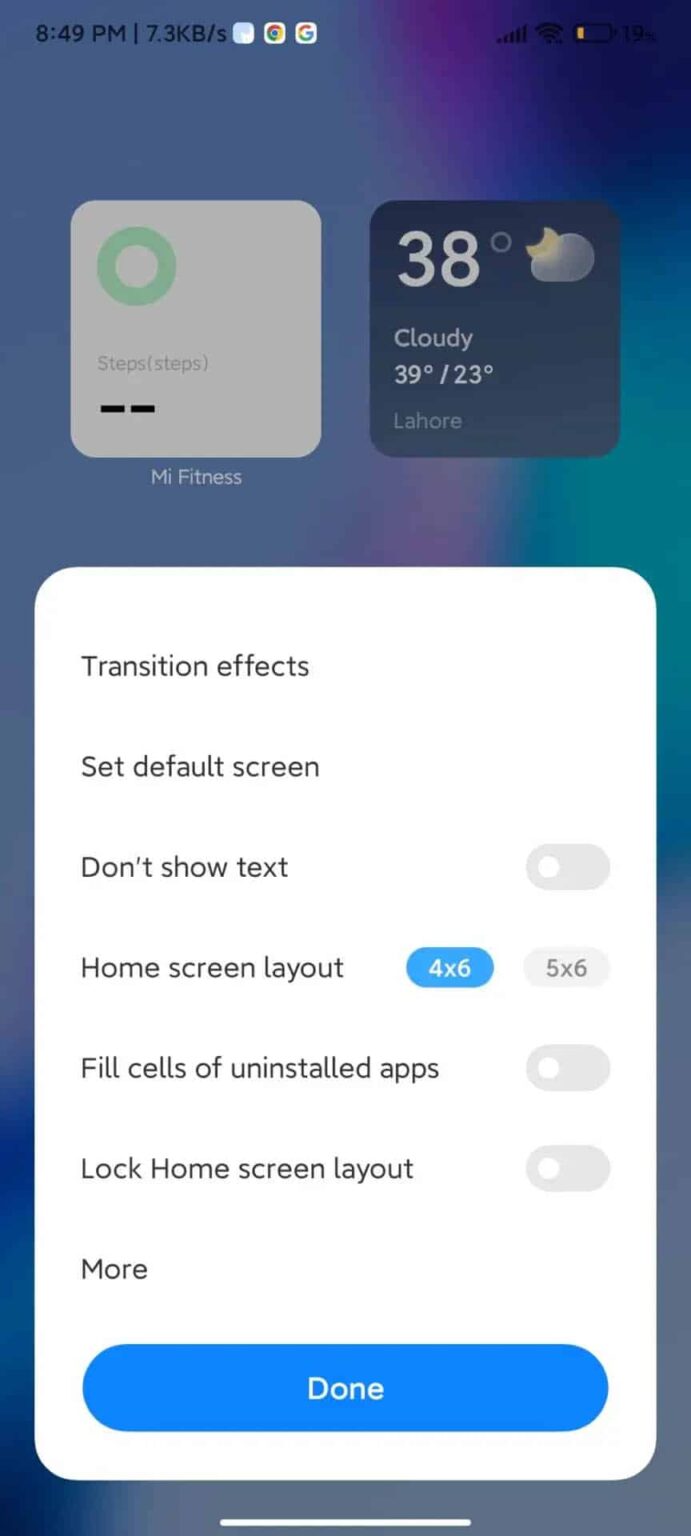This is a detailed screenshot of an iPhone home screen. The time at the top reads 8:49. The battery is notably low, but it's partially obscured by a dark purplish overlay in the top-right corner, making the exact battery percentage indeterminate. Prominently displayed is a "MyFitness" widget, which usually tracks steps, but currently shows no recorded steps.

The weather widget indicates it is 38 degrees Fahrenheit and cloudy in Lahore. The settings menu is open, showcasing options such as transition effects and home screen layout. The background is plain white, and there is a blue "Done" button available for selection at the bottom of the screen.